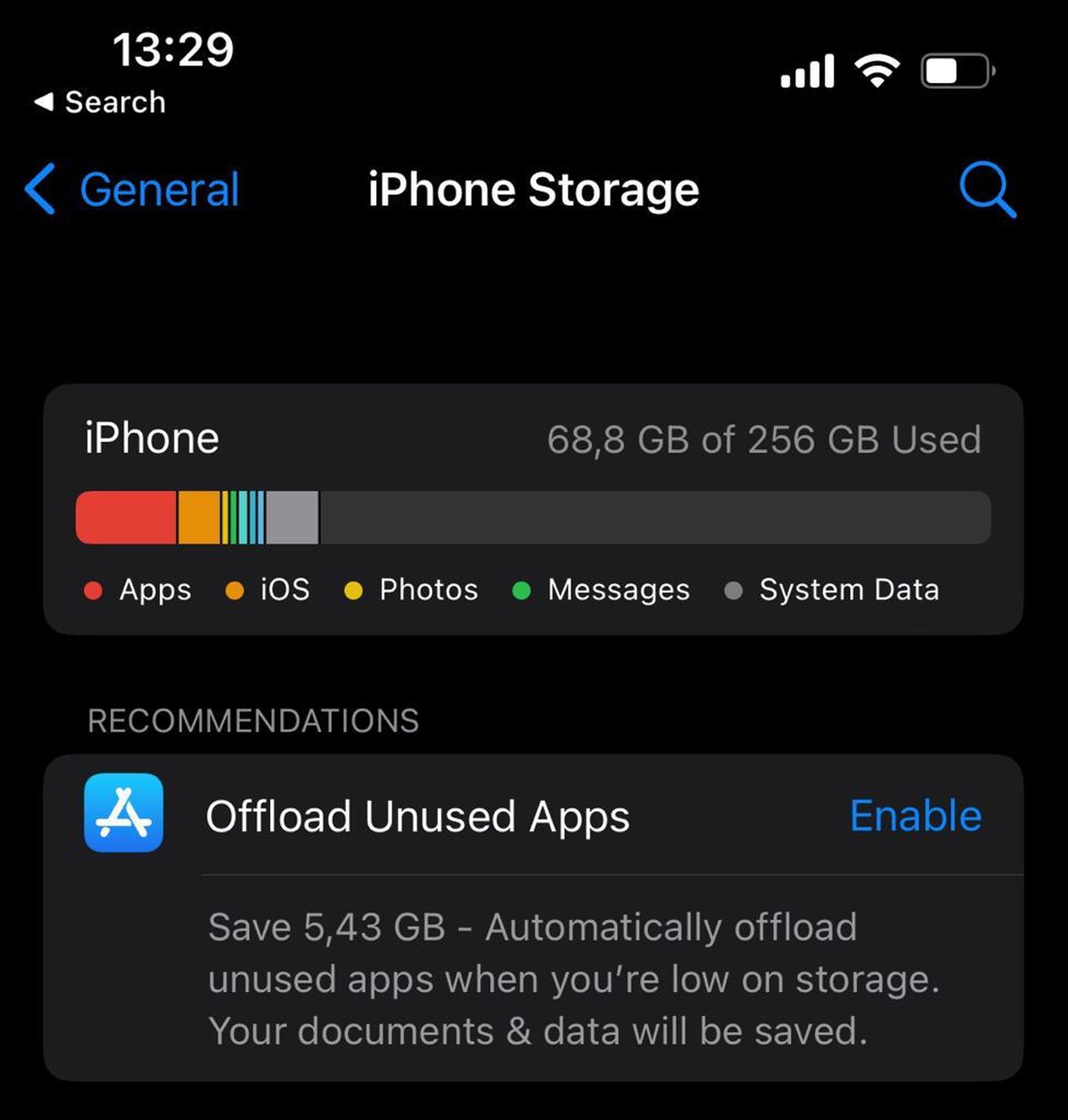The screenshot of the iPhone storage interface displays various informational elements that provide a snapshot of the device's current data usage. At the top left corner, the time reads 13:29, while the top right corner shows the signal strength with four bars, Wi-Fi connectivity, and a slightly depleted battery icon. 

The center of the screen prominently features the title "iPhone Storage," with a "General" tab captioned to the right and a back arrow pointing left. A search icon is positioned to the far right, indicating the function to search within the storage settings.

Below this header, a detailed storage bar graph illustrates the distribution of the iPhone's used space. The graphical representation specified 68.8 GB used out of a total 256 GB capacity. The bar is segmented into colored sections: a red section representing apps, which is the most substantial portion, a gray section signifying user system data, and a smaller yellow section indicating space taken up by the iOS system. Each color-coded section correlates with labels that assist in identifying what categories are consuming the storage capacity.